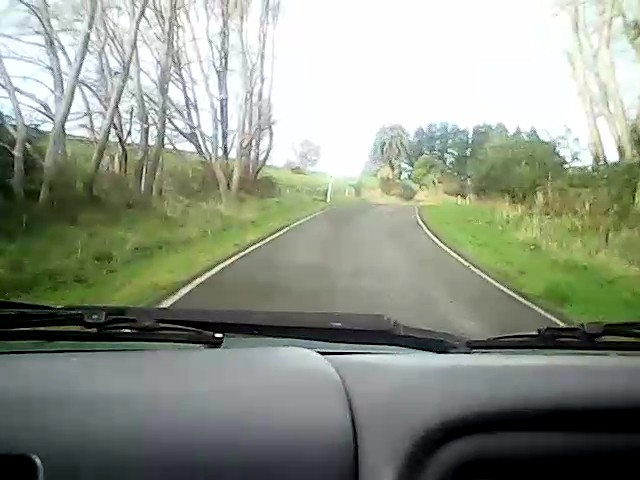The color photograph is taken from the interior of a car, offering the driver's perspective through the windshield. The scene ahead shows a narrow, single-lane paved road, possibly a driveway, bordered by white lines. On either side of the road are grassy fields, adorned with several trees, likely birch trees, given their light-colored trunks and absence of leaves. The image is slightly blurry, making it difficult to clearly distinguish certain details, but in the distance, a disturbance on the road is visible, possibly an animal, like a bull, or a natural event such as flooding, an earthquake, or a landslide. The horizon shows a line of fuller, greener trees under a bright yet overcast sky, adding to the serene yet mysterious atmosphere of the photograph. The dashboard is also partially visible, emphasizing the in-car viewpoint.